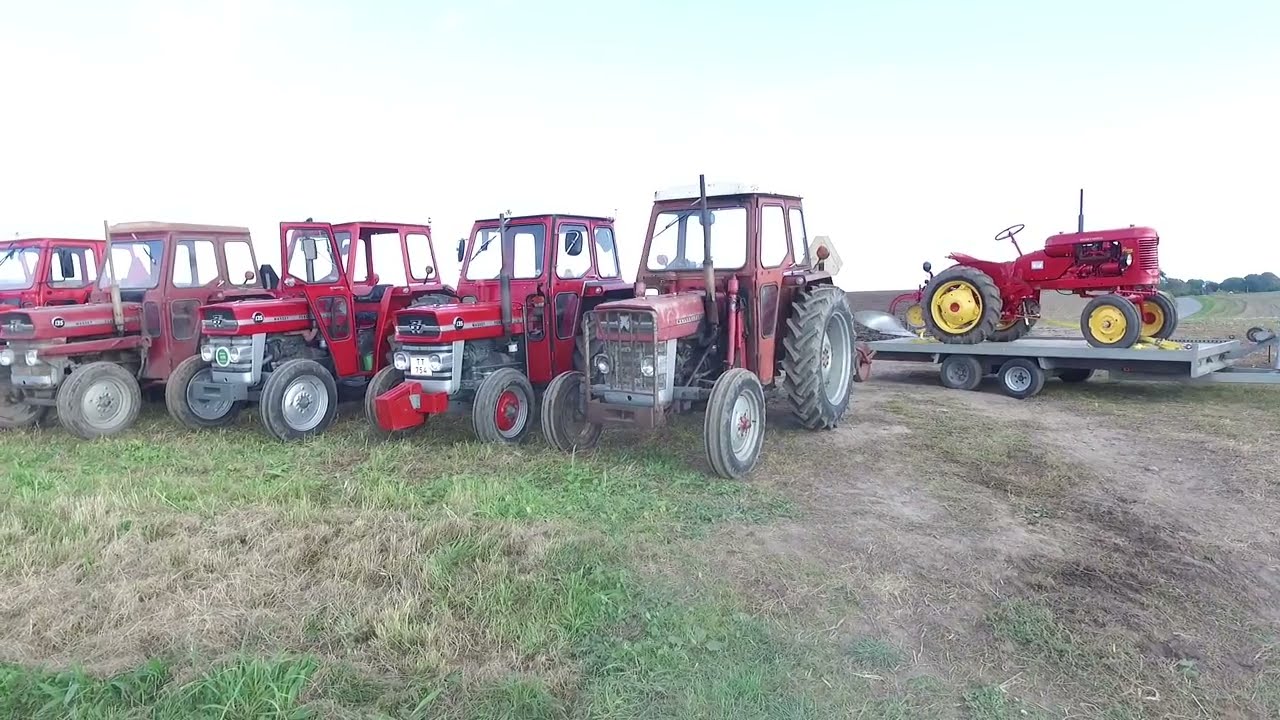The image depicts a row of five red tractors diagonally parked from the center to the left side, each with cabs in varying shades of red, some featuring grey accents. On the right side, a single red tractor with yellow rims sits on a grey metal trailer, equipped with black rubber tires, dual small wheels on each side, and a curved silver fin blade plow at the back. The scene is set outdoors in a field, characterized by a blend of green and light brown dry grass, with patches of soil visible in the bottom right corner. The sky is a light white, indicating daytime conditions, and the background features a grey road and green trees. The tractors, all featuring black wheels and lights, are positioned on mostly dry grass, suggesting a warm climate.